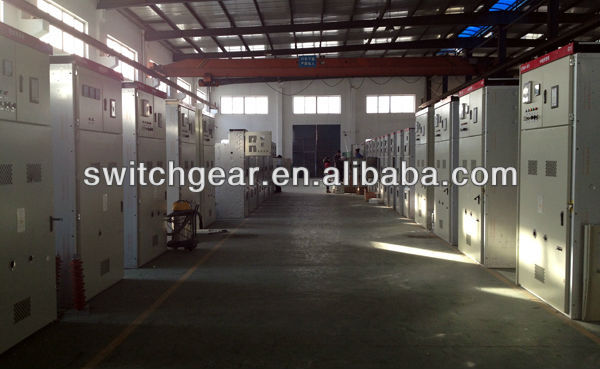This detailed photograph captures an industrial setting, likely within a factory or a power facility. The room exudes a distinctly utilitarian and somewhat stark ambiance, characterized by its concrete floor and dark, muted color palette. Centered prominently across the image is the text "switchgear.en.alibaba.com," suggesting a reference to electrical equipment.

Spanning the length of the room, a wide walkway is flanked by rows of towering grey cabinets or lockers, which are lined up in parallel on each side. These cabinets, each approximately 7 to 8 feet tall, feature maroon red tops and various buttons, indicative of electronic or network equipment rather than mere storage. The equipment-filled hallway continues seemingly endlessly, as more cabinets disappear into the distance.

Natural light filters through small windows near the ceiling, casting shadows that subtly break the room’s monotone appearance. Towards the back of the room, a few people can be seen standing near a doorway, engaged in conversation, adding a small touch of human presence to the otherwise mechanical environment.

Above, the ceiling is constructed from a material resembling translucent plastic or porcelain glass, supported by a framework that appears to be crisscrossed wood or some other supportive structure. Additionally, a shop vacuum, identifiable as a "shop vac," is positioned near the center of the room, highlighting the ongoing maintenance and industrial activity within this space.